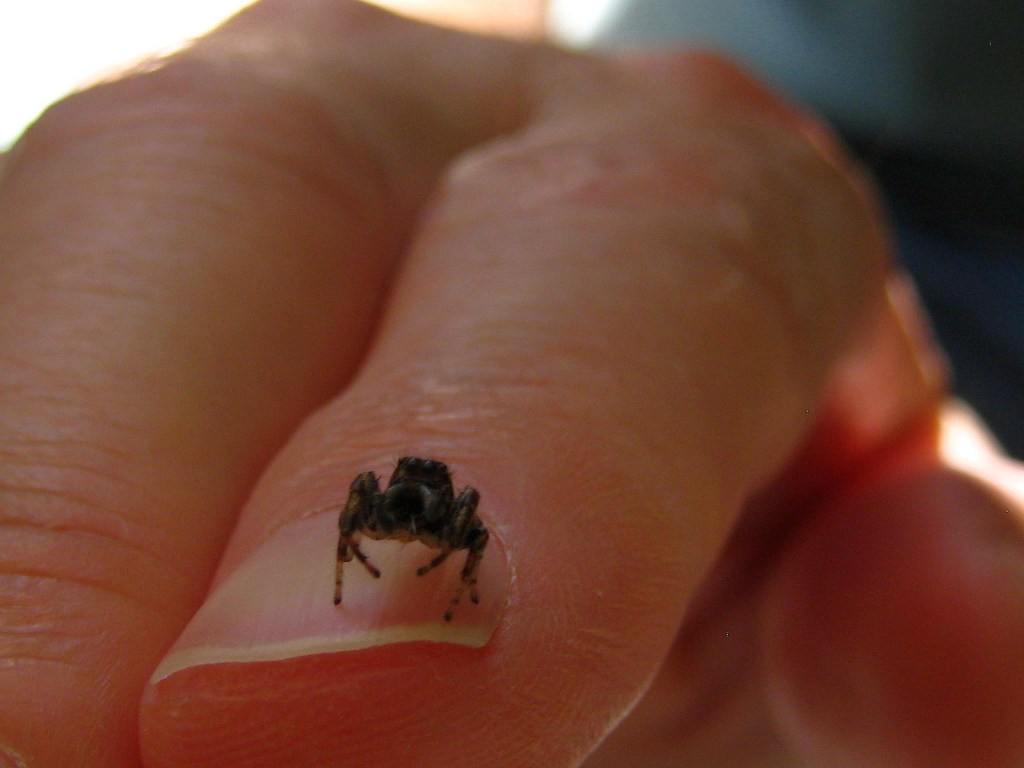This extremely close-up, rectangular photograph depicts a light-skinned human hand, focusing on the index and middle fingers with the thumb just visible at the side. The well-groomed, short fingernails dominate the foreground, with a black and yellow spider perched on the nail of the index finger. The spider, facing toward the camera, displays at least five legs, with some raised. The skin texture and knuckles are slightly visible, and the background is softly blurred, revealing a hint of a blue-green shirt. The top corners of the image feature a contrasting light spot to the left, likely from a light source, and a faded black area, possibly the person's chest or shirt, in the top right.